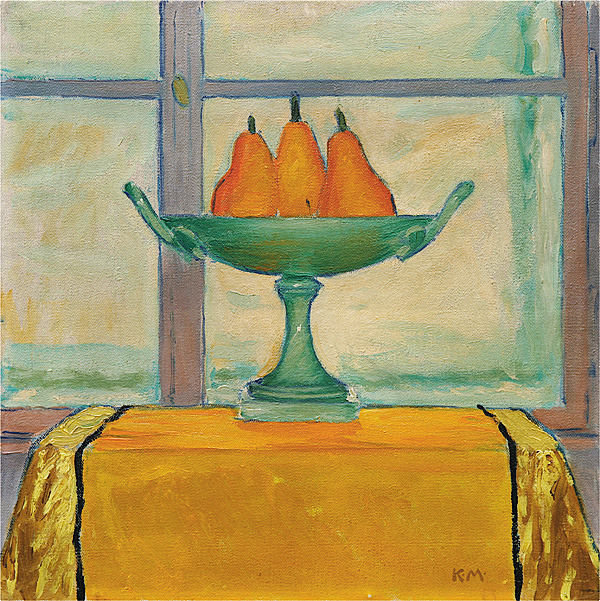The painting, bearing the initials KM in the lower right corner, likely a watercolor, depicts a simple yet elegant still life. Central to the scene is a table draped with a gold tablecloth, the edges of which are a lighter shade of yellow and separated by a black line. Atop the table sits an aqua turquoise pedestal bowl containing three upright pears, with the middle pear being the tallest. Behind the table, a window with purple trim and a gold latch splits in the middle, its two panes opening outward. The window offers a softened, indistinct view of the outside, featuring a blend of yellowish and cream hues with faint green streaks. The overall composition, with its understated yet harmonious use of color, suggests it might be the work of a beginning art student.